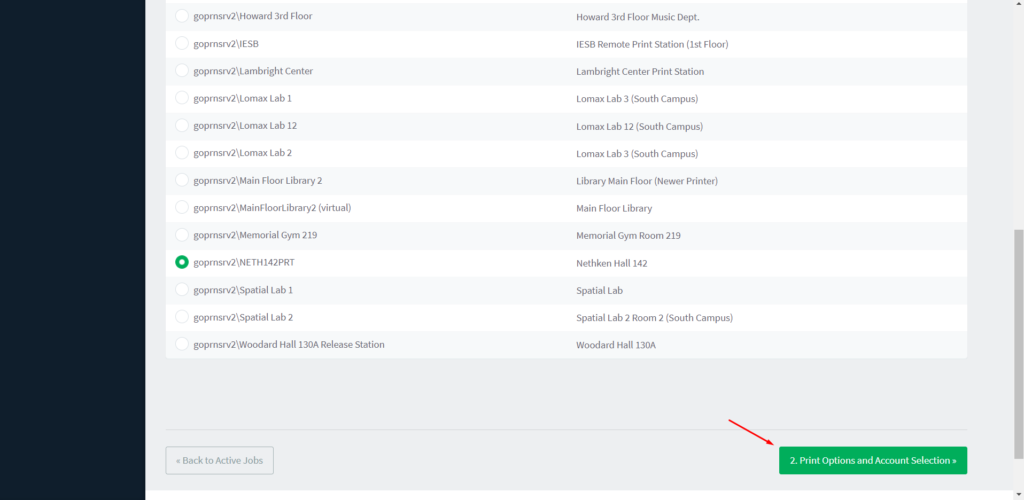This image is a screenshot of a list that appears to detail various printing locations within a college campus. The list is neatly organized with alternating gray and white rows to enhance readability. On the left of each row, there is a selectable radio button. The far-left column remains blank, separating the list from the rest of the interface. Each entry consists of a location name followed by a detailed description:

1. **Howard 3rd Floor** - Identified as the Music Department.
2. **GOP RNS RV2 ESB** - Designated as the Remote Print Station on the first floor.
3. **GOP RNSV2 Lambright Center** - Specified as the Print Station at Lambright Center.
4. **Lomax Lab 1, Lomax Lab 2, Lomax Lab 12** - Each listed with corresponding labs.
5. **Main Floor Library 2** - Described as the Library Main Floor Newer Printer.
6. **Main Floor Library 2 Virtual** - Indicated as the Virtual Printer on the Library Main Floor.
7. **Memorial Gym** - Located in Room 219 of the Memorial Gym.
8. **NEF 142 PRT** - Situated in Nefkin Hall 142.
9. **Spatial Lab 1, Spatial Lab 2** - Printers available in these respective labs.
10. **Woodard Hall Release Station** - Found in Woodard Hall Room 130A.

This organized structure allows users to easily find and select their desired printing location across the campus facilities.